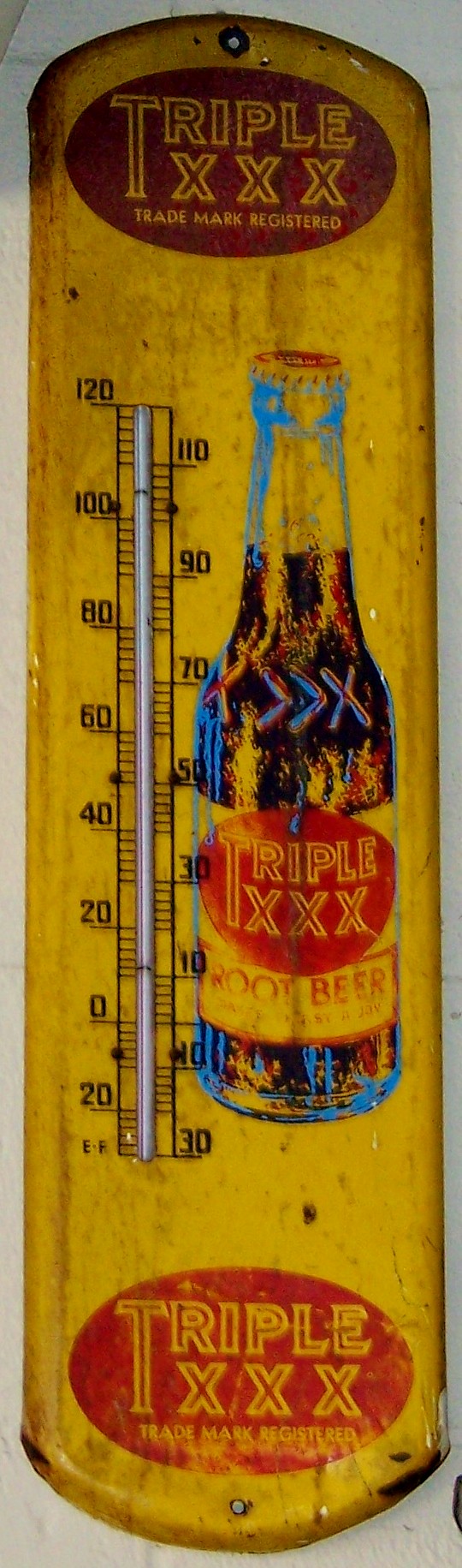This image features a vintage metal thermometer with a notable yellow finish that's aged over time, exhibiting numerous brown rust marks and stains. The thermometer is vertically oriented, displaying signs of extensive use. At the top of the thermometer, there's an oval-shaped marking in a dark red shade, featuring the text "Triple X Trademark Registered" in yellow. A similar oval bearing the same text appears at the bottom, though it's in a brighter red hue.

The center of the thermometer showcases a classic bottle of Triple X Root Beer, distinguished by its clear glass exhibiting blue, brown, and red details, and containing a dark brown liquid. To the left of the bottle is the temperature gauge, which has a scale ranging from 30 degrees to 120 degrees Fahrenheit. For easy mounting, the thermometer is equipped with two holes, positioned at the top and bottom, suitable for screws or nails.